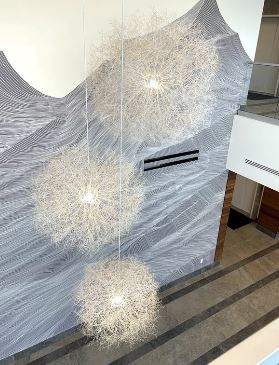The picture, taken from a higher perspective, showcases an art exhibit or decorative installation featuring three grayish-white light fixtures suspended from white strings. These lights, resembling fiber-optic tumbleweeds or puffy dandelions, hang in front of a grayish-blue painted wall that adds a modern aesthetic to the display. The installation appears to be set inside a professional building, possibly a school or office, with a polished wooden or brown-striped floor. The photograph captures a high-angle view, suggesting the photographer stood on a second floor, overlooking the exhibit on the lower level. The goal of this setup seems to highlight the contrast between the intricate, delicate lights and the neutral, textured background.